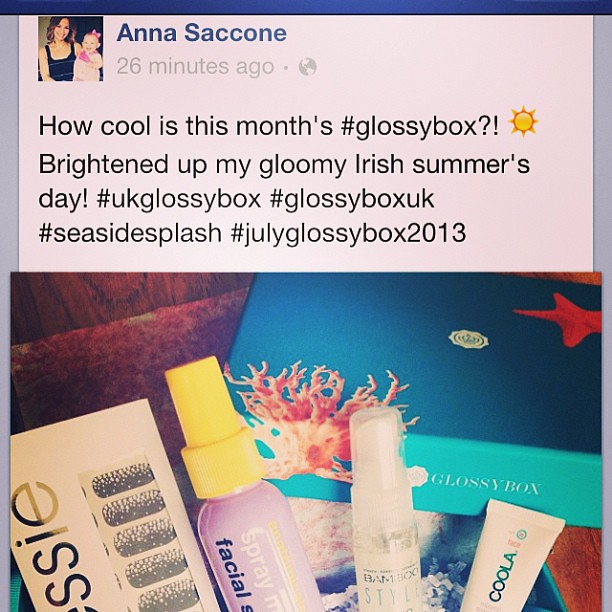Anna Saccone posted publicly 26 minutes ago: "How cool is this month's Glossy Box? 🌞 Brightened up my gloomy Irish summer's day. #UKGlossyBox #GlossyBoxUK #SeasideSplash #JulyGlossyBox2013." 

The post includes a photo of an open Glossy Box adorned with ocean-themed illustrations like sea stars and anemones. Four visible items are fanned out from inside: a facial cream in a pink container with a yellow top, a transparent bottle likely containing liquid moisturizer, a product labeled “COOLA” in blue letters, and another partially visible item. The blue Glossy Box itself has coral-like designs in yellow and rust-colored stars, with "Glossy Box" written in white on the side.